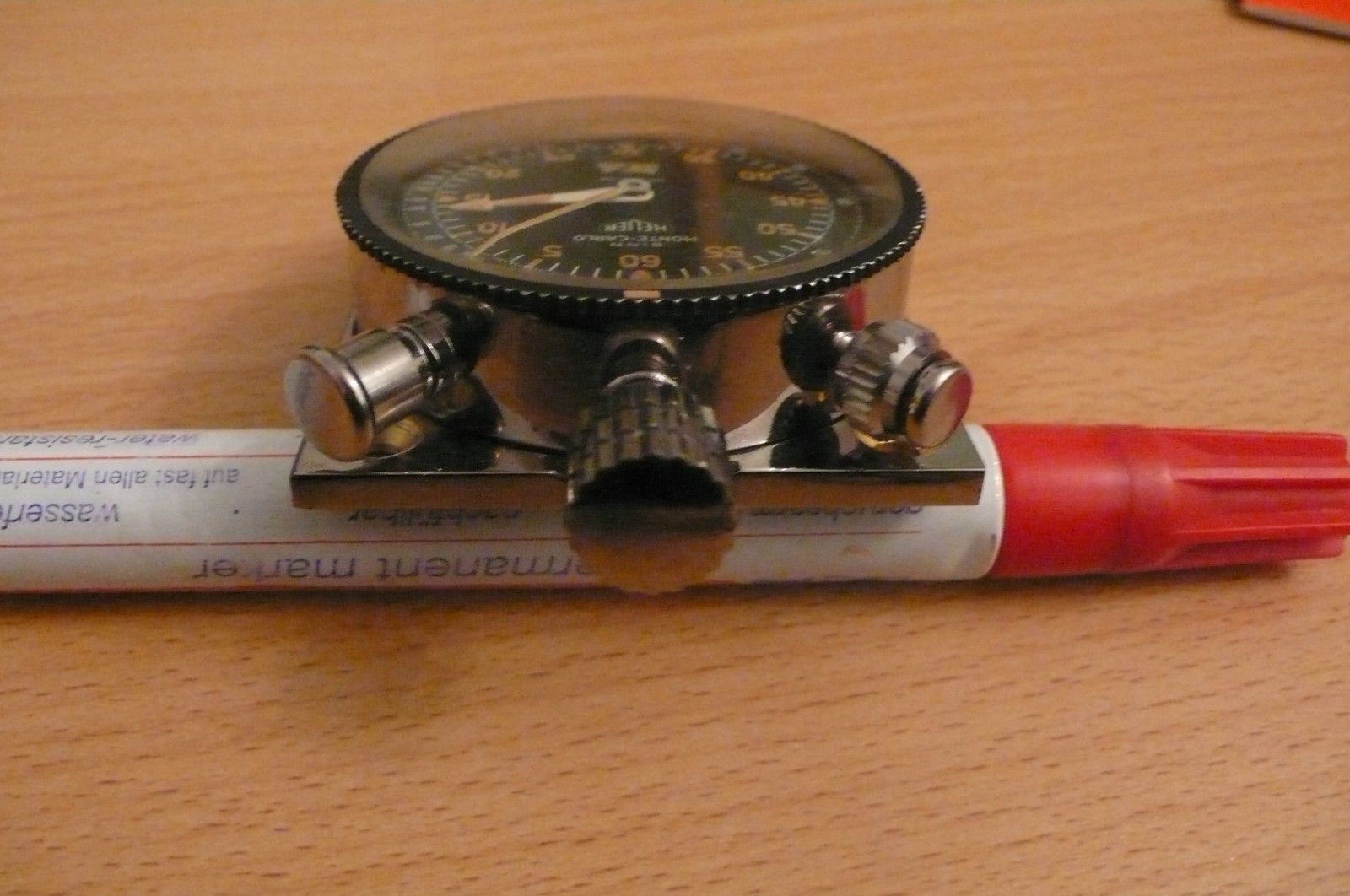In this image, a light wooden table serves as the backdrop. Positioned in the upper right corner, a red notebook is partially visible. The main focus of the photo is a red permanent marker with a white body, adorned with blue text that reads "Permanent Marker," alongside some German writing that includes the word "Allen," suggesting the photo may have been taken in Europe. Leaning against the marker is a vintage-style mini timer, featuring a silver frame and a black interior with numeric markings up to 60. The timer has a traditional alarm clock appearance with a winding button on top and two side buttons. Currently, the timer's larger hand points to 14, while the smaller hand rests on 8. The timer is supported by a square base, and its old-fashioned design suggests it might be used for a specific timed activity or project.